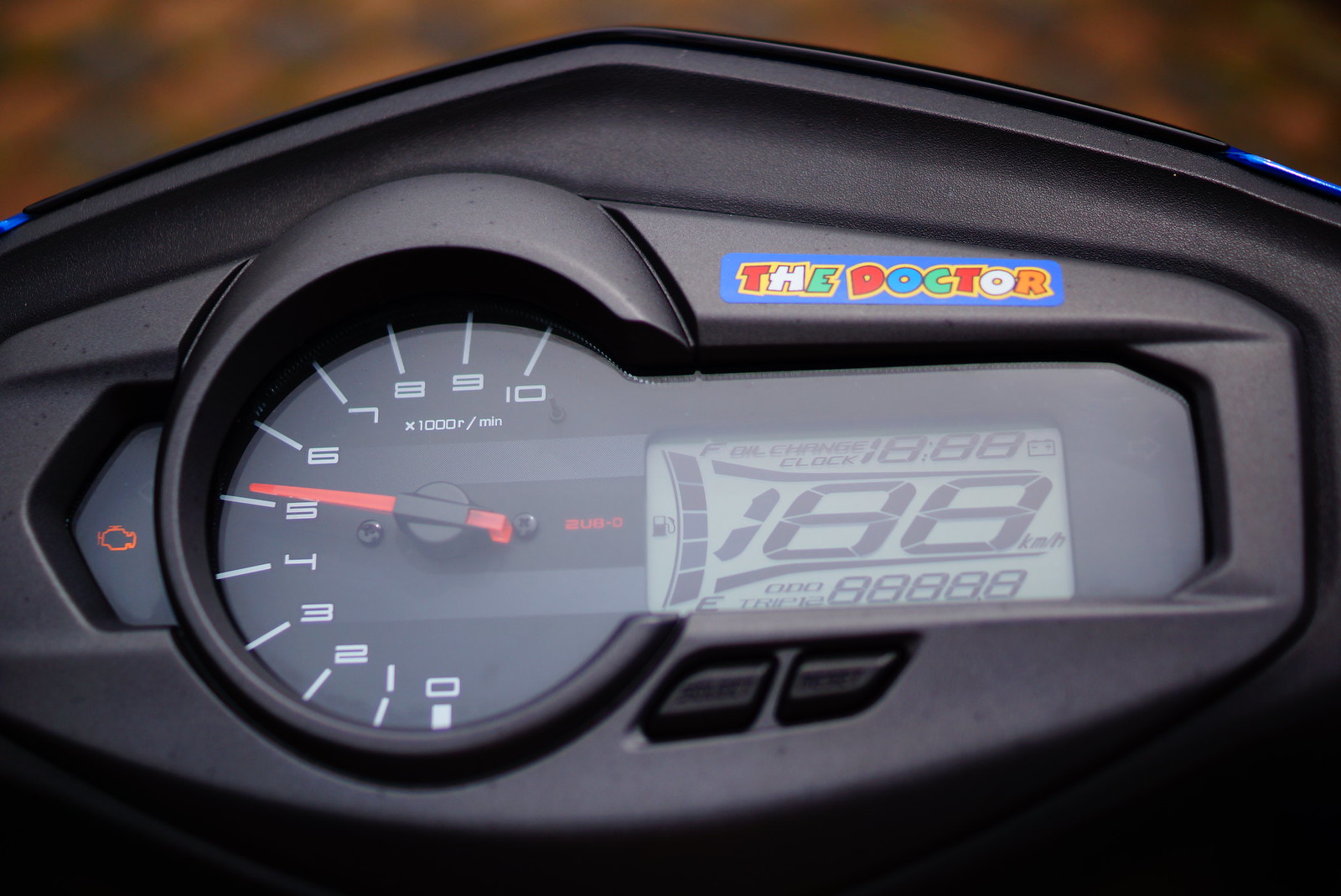The image displays an intricate dashboard of a game console adorned with a sticker that reads "The Doctor." The console's digital screen is illuminated, showcasing an array of information. Prominently, the display shows a speed indicator with a zero reading, alongside a digital clock labeled "Oil Change," which currently reads "188." A gas pump symbol indicates a full tank, with all the fuel markers lit.

Adjacent to the gas indicator is a dial encompassing a range from 0 to 10, marked "times 1000R over MIN." The red needle of the dial, held by a black fixture, points precisely at zero and is connected to a central cylinder. A red text, "2UB/0," is also displayed on the screen.

To the left of the dial, a check engine light is illuminated, signaling potential engine issues. Beneath the right side of the console, two buttons are visible, though their labels are illegible in the image.